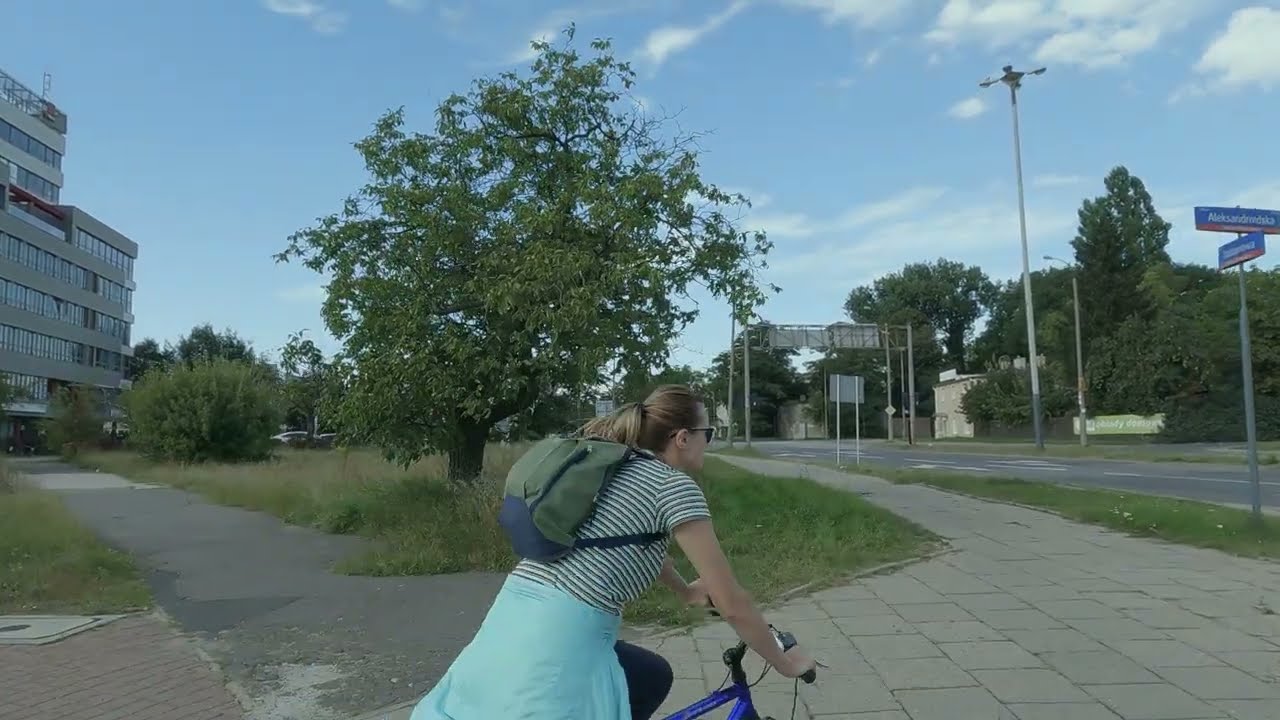A horizontally aligned, rectangular photograph captures a woman riding a bicycle on a brick-paved pathway in an urban setting. The woman, seen from behind, has dark blonde to brown hair neatly tied in a ponytail and wears black sunglasses. She sports a short-sleeved, green and white striped t-shirt, black pants, and a light green or turquoise jacket tied around her waist. A green backpack with visible straps is secured on her back. She rides a royal blue bicycle with black handlebars, of which only the front part is visible in the frame.

In the center of the image stands a large tree, and the path she is on is lined with well-worn, large square bricks. To the left of the path lies a cracked, smaller road bordered by tall grass and more trees. A multi-story building, resembling a brownstone with numerous windows, can be seen behind the road. On the right side of the image, there’s a street with traffic signs—blue rectangles with foreign text—and streetlights. The sky above is mostly blue with wispy white clouds, and beyond the tree is a green grassy field interspersed with additional trees and shrubs.